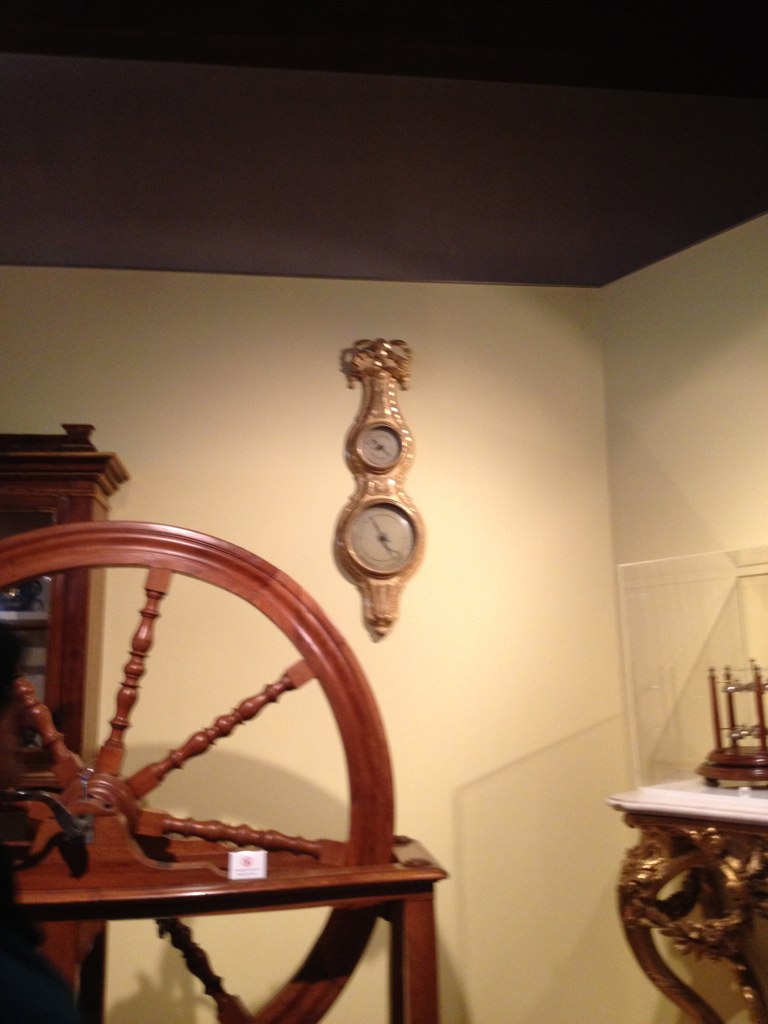The photograph captures an elegantly decorated room with a focus on antique furnishings. Prominently displayed on the ivory-colored back wall is a large, ornate gold clock featuring two faces, reminiscent of a corn husk texture. The upper part of the clock displays a smaller face, while the lower section showcases a larger timepiece, though the times are not discernible due to the distance. In the foreground, a giant antique wooden wheel rests inside a narrow wooden table, adding a sense of historical charm. To the lower right, an exquisite antique golden table with a white marble top further enhances the period aesthetic. The ceiling above contrasts with the walls in a rich brown hue, adding depth and warmth to the scene.